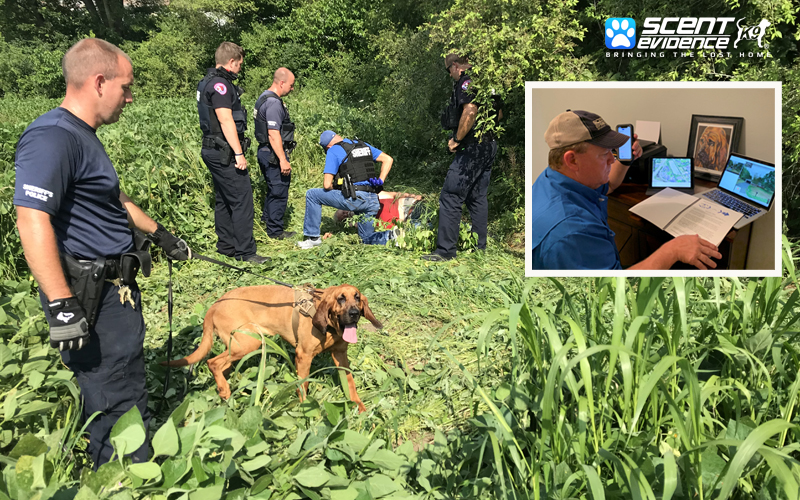The main image captures a group of police officers in a dense, grassy patch of a forest, likely engaged in a search operation. There is visible lush green vegetation, including tall grasses and trees, as the officers stand under a sunny sky. The foreground features a police officer in a t-shirt and blue pants, handling a brown bloodhound on a leash, which has its tongue sticking out. The officer, equipped with fingerless gloves and a sidearm, appears to be a canine handler. In the background, more officers in navy blue uniforms, some with "Sheriff" vests, are gathered, with one officer kneeling possibly over a body, suggesting this might be a real search or a training exercise. The inset image in the upper right corner shows a man in a blue shirt and baseball cap holding a phone, surrounded by a tablet, laptop, papers, and a photo of a dog, hinting at coordination and tech-savvy support. A watermark at the top right of the main image reads "Scent Evidence, Bringing the Lost Home," accompanied by a blue icon of a white paw print and another icon that reads "K9".